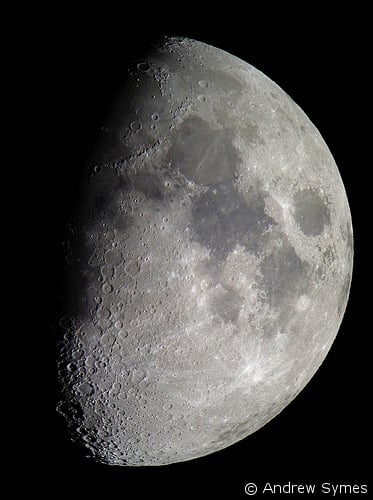This detailed photograph captures the moon in a stunning close-up, revealing intricate surface details including craters, light and dark gray splotches, and reflective flecks. The image is composed in a rectangular format, where approximately three-fifths of the moon is visible; the remainder is cloaked in shadow. The illuminated portion of the moon's surface contrasts sharply with the blackness of the background, devoid of any stars, enhancing the prominence of the lunar features. The photograph's bottom right corner displays a copyright mark followed by "Andrew Symes" in white letters, indicating ownership. The intense focus and high level of detail suggest that this photo may have been taken from space, offering a spectacular and immersive view of the moon.